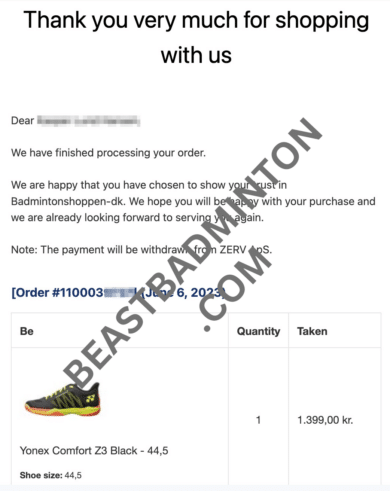This image displays a confirmation message on a smartphone screen, originating from a webpage. The background is white with the text in black print. At the top, it reads "Thank you very much for shopping with us." Following this, the message addresses the customer directly, though the name and personal information have been blurred out for privacy.

The message continues, "We have finished processing your order. We are happy that you have chosen to show your trust in Badminton Shoppers - DK. We hope you will be happy with your purchase and we are already looking forward to serving you again. Note: The payment will be withdrawn from Zerve/OS."

Further down, the order details are partially visible. The order number and some related information are blurred out, but the date "June 6, 2023" is clear. The seller's website "beastbadminton.com" is listed, along with the order specifics:

- Quantity: 1
- Price: 1,399.00 KR

The product description states "Zonix Comfort Z3 Black 44.5" with the shoe size noted as 44.5.